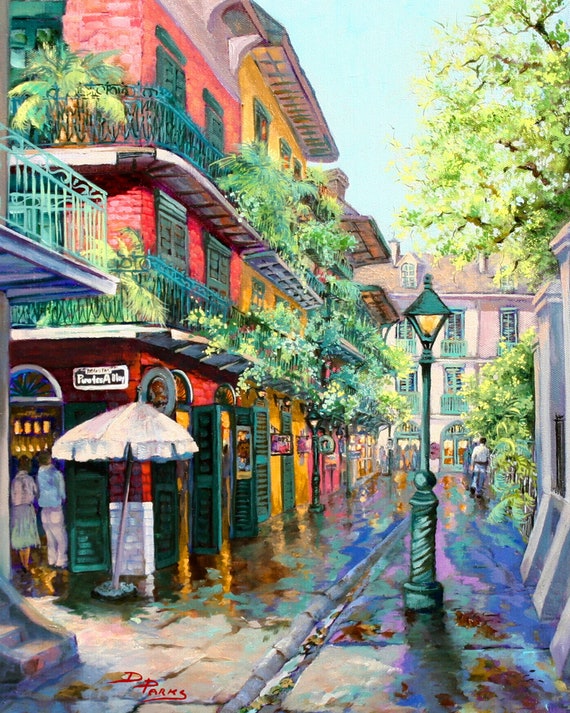The image depicts a vibrant street scene with an illustration on the sidewalk in the foreground, made up of gray and brown hues. The illustration is signed "D. Palms" in red lettering, suggesting it was created by this artist. The sidewalk extends from the foreground to the background, leading towards a white building. On the right side of the image, a black streetlight stands prominently. The left side features an array of colorful buildings: a tall red building, followed by a tall yellow building, another red building, and finally, a white building. Each building is adorned with green metal terraces and window frames in a bright green color, adding to the lively atmosphere of the scene.